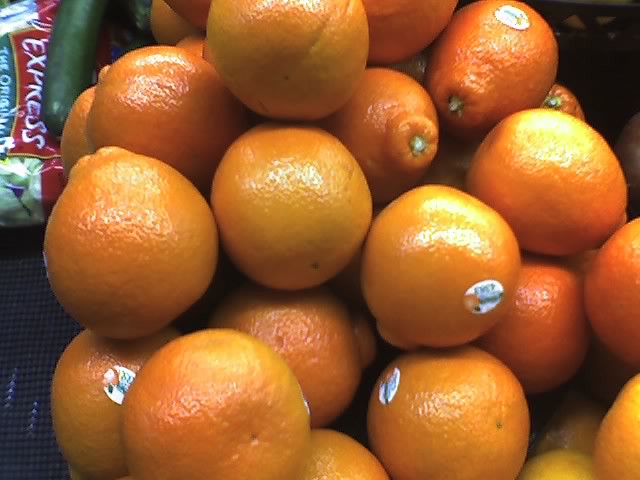The image displays a vibrant and neatly arranged pile of oranges, approximately 15 to 40 in number. The oranges are stacked closely together, showcasing their round, mostly uniform shapes with some slight irregularities. They are of moderate size and exhibit a bright, ripe orange hue, though some vary from darker to lighter shades. Most of the oranges feature small, oval stickers with orange and white colors, possibly indicating their origin, evoking a "Florida" look.

In the upper left corner of the image, just behind the oranges, there is a partially visible bag of salad. The salad bag prominently features the word "express" and the phrase "the original" in white text on a green background. You can peek through the bag to see some lettuce and purple cabbage. Resting atop the salad bag is a cucumber. The backdrop and the mat blacks suggest the setting might be a grocery store or a produce haul displayed on a kitchen counter. The photograph is taken up close, emphasizing the size and details of the oranges while leaving the salad bag and cucumber partially out of focus. The upper right corner of the image is shaded, contrasting with the bright oranges.